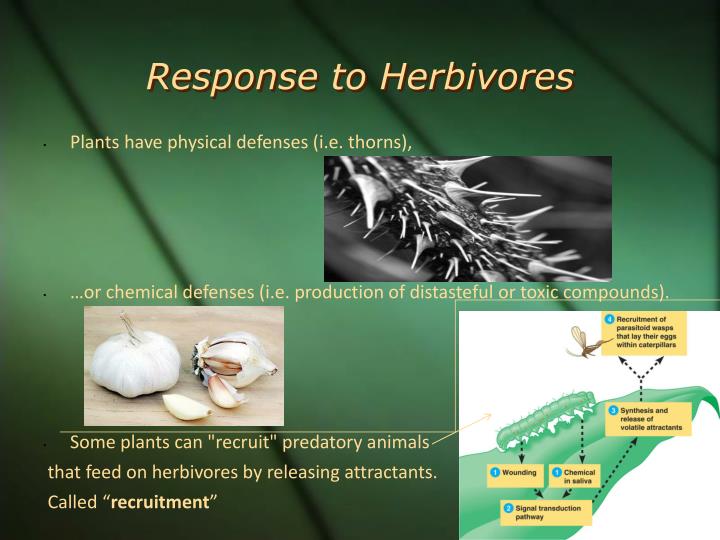The infographic presents a detailed guide on plant defenses against herbivores, set against a dark green background. Across the top, in large, slightly italicized light yellow lettering, it reads "Response to Herbivores". Below this, it elaborates on plant defenses, starting with "plants have physical defenses (e.g., thorns)," showcased by a black and white photograph of a thorny stem angled at 45 degrees. This photograph is positioned on the upper right side but not fully edge-to-edge.

Beneath this, the infographic continues with "...or chemical defenses (e.g., production of distasteful or toxic compounds)," highlighted by a light brown inset featuring a whole head of garlic and some broken cloves. Following this section, in yellow print, is text explaining that "some plants can 'recruit' predatory animals that feed on herbivores by releasing attractants called recruitment."

In the bottom right corner, set against a white background, a detailed flowchart illustrated with a light green leaf and a caterpillar, likely being preyed upon by a drawn insect. This section includes five gold rectangular boxes with black descriptive text and arrows indicating interactions, though the specific text in the boxes is unreadable. Each gold rectangle features a blue icon in the upper left, possibly indicating additional information or steps.